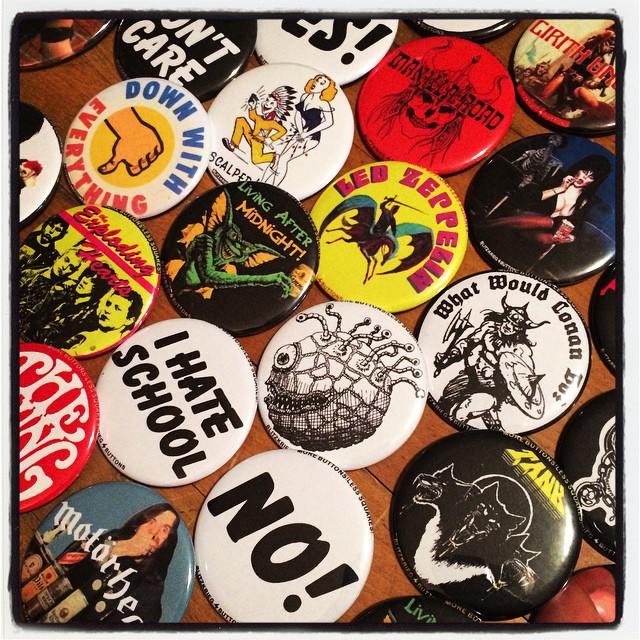The photograph showcases a collection of vibrant and eclectic pin-on buttons meticulously arranged on a brown wooden table made of diagonal boards, stretching from the bottom right to the upper left corner. Among the myriad of buttons, there are noticeable rows with various themes and striking designs. The top-most visible row features a red button with a skull adorned with long hair. Adjacent to it is a darker button displaying an image reminiscent of Elvira, the iconic vampire lady. Following this is a notable white button with the phrase "I hate school" and another one with a loud "NO!" in big black letters. Additionally, there’s a fascinating pin depicting what looks like a glamorous pinup figure, possibly inspired by Marilyn Monroe, alongside a button featuring a stereotypical Native American figure. Another distinctive piece is a yellow button with bold red lettering saying "Led Zeppelin" circling the top, showcasing a figure riding a pegasus, brandishing a sword mid-flight. Complementing this is a pin that proclaims "What Would Conan Do?" with an image of Conan the Barbarian in monochrome. The collection includes various other pins with expressions like "Down with everything" accompanied by a thumbs-down symbol, and one highlighting the band Motorhead with an image of its musician. The vibrant assortment of pins, ranging in colors from white, black, red, to yellow, collectively present a rich tapestry of pop culture and iconic imagery on the rustic surface of the wooden table.